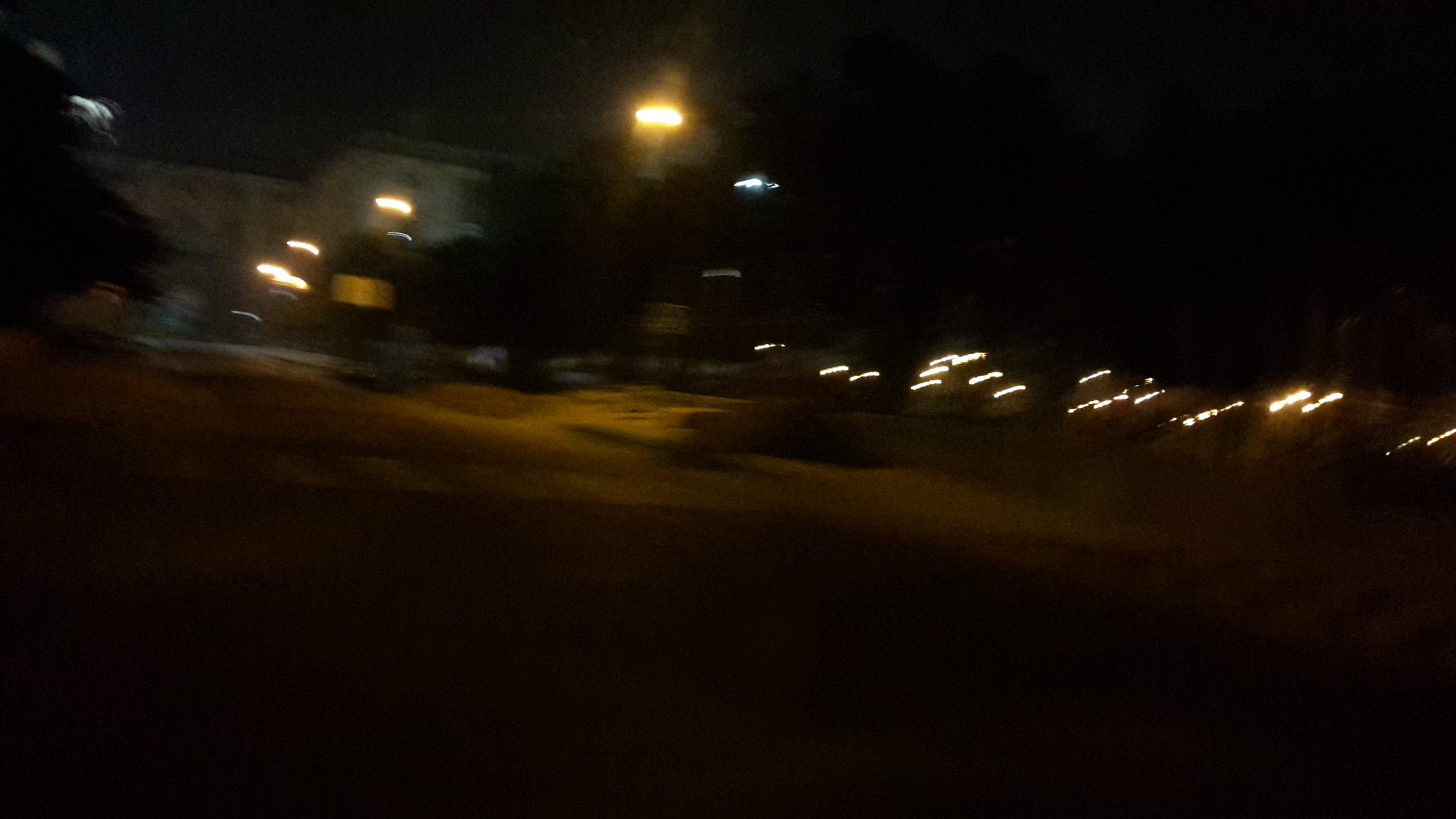The image depicts a nighttime scene captured from a moving car, resulting in significant blurriness. The photograph features a white, two-story house in the background. This house is partially obscured by dark-colored trees, which are only silhouettes due to the nighttime conditions. A prominent yellow streetlight illuminates the scene, casting a yellowish glow onto a green lawn. There is one noticeable window in the house that is lit with a yellow light, while other windows remain dark or indistinguishable. The blurred motion has transformed various light sources into curved lines, and a set of these lights appear to be car headlights. Additional lights are visible in the background, possibly hinting at taller buildings or other structures. Towards the top right, the image is dominated by a dark night sky. Scattered throughout the photo are white lines caused by the camera's movement, and the foreground remains an indistinct, gray blur. A yellow sign and another tree can be seen on the left side, adding more layers to this blurry, chaotic nighttime shot.